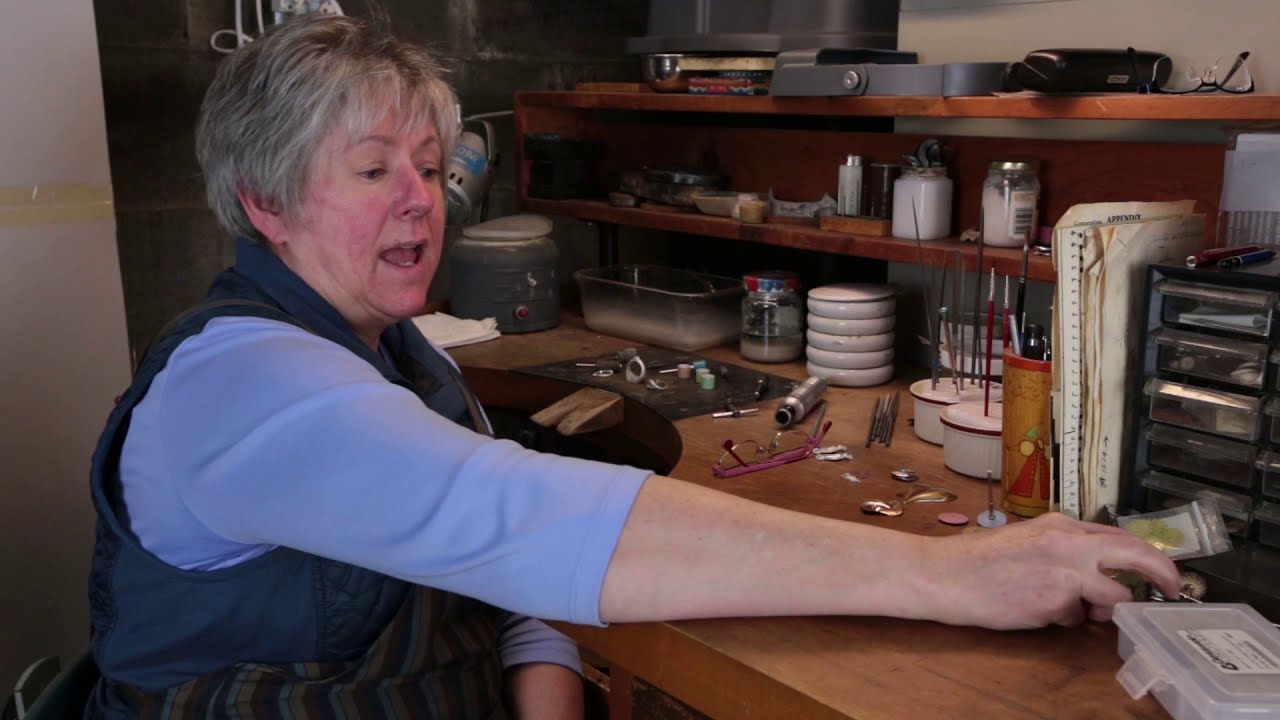An elderly Caucasian woman with short gray and black hair sits at a large wooden work desk. Dressed in a light blue shirt that extends to her elbows and a darker blue vest, she is engaged in a crafting activity. The desk, positioned to her right, features shelves built into its back section, cluttered with various craftsmanship materials. Her right arm is outstretched, reaching toward a silver plastic bag containing a gold item on the desk's surface. Scattered around are several items including small cups with paintbrushes, a white cylinder with ripples and a top, jars, and a plastic container with a white label in the bottom right corner. Ordinarily seeking details, she gazes slightly down and right, as though speaking or explaining her craft, with a small portion of her teeth visible as her mouth is slightly open. The scene evokes a meticulous and intimate workspace dedicated to intricate handiwork, possibly involving buttons and painting supplies.